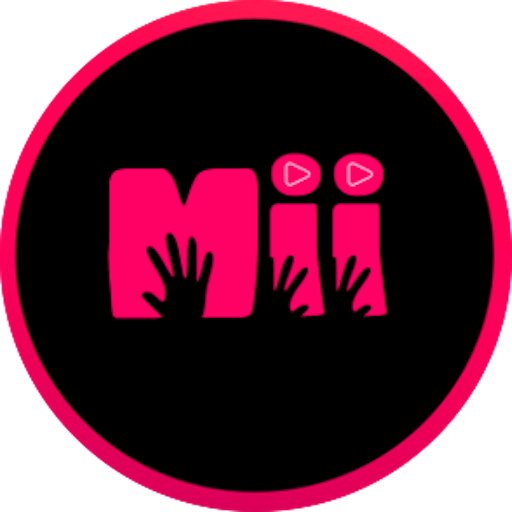The image features a prominent circular design with a narrow, red frame. Within this frame, the background is black, creating a stark contrast. Centrally positioned within this black interior, bold red letters spell out "ME," with an alternative interpretation of "M-I-I." Unique to these letters, the dots above the "I"s are depicted as the YouTube logo, featuring play buttons. Silhouettes of human hands in black are intricately integrated into the design, appearing as shadowy cutouts in front of the lettering. The image's color scheme includes shades of red, black, and white, giving it a striking visual appeal. The overall setting suggests this could be an advertisement for a product or service, emphatically branded as "ME."